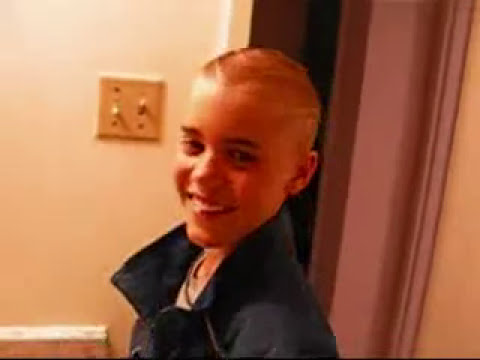In this image, we see a young person with a very short, almost shaved haircut reminiscent of a buzz cut, smiling warmly. Their eyes are a dark color, possibly brown, and they have a light gray t-shirt on underneath a navy blue jacket with a large collar. The person, who could be a young boy or girl, is standing in what appears to be a brightly lit room, possibly a bathroom, given the white walls. Behind them, there is a slightly dirty, double ivory light switch and a doorway with a folding door that appears to be a light or pastel pink. The close-up shot captures the person from the shoulders up, and they are looking slightly below and to the left of the camera, giving the impression of a candid, almost lively smile.